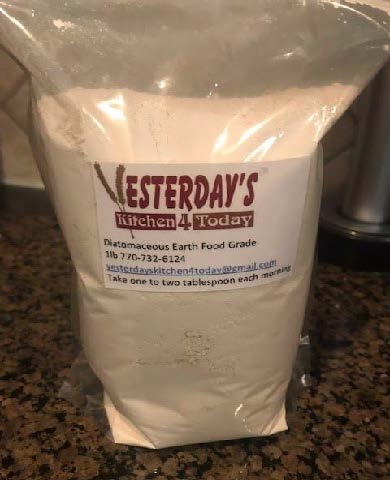The photograph captures a large plastic bag placed on a tan stone countertop, speckled with large black fragments, in a kitchen with a white wall in the background. The bag, which is tightly sealed with a zip top, is filled with a white powder, occupying approximately four-fifths of its volume. Prominently displayed on the front of the bag is a white label with red and black text. The red text reads, "Esther Day's Kitchen for Today." In smaller black text, the label details the contents as "Diatomaceous Earth Food Grade, 1 pound," followed by a contact number "770-732-6124" and an email address, "Esther Day's Kitchen for Today at gmail.com." The label also includes usage instructions, recommending taking "1-2 tablespoons each morning." Despite minor discrepancies in the image descriptions, it is evident that the product is likely intended as a nutritional or supplemental powder.